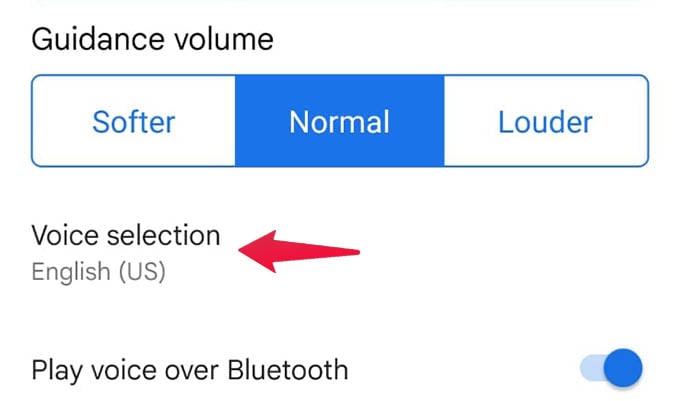The image is a screenshot of a phone's settings related to audio guidance. At the top left, the header "Guidance Volume" is displayed in black text. Below this header, there is a rectangular slider divided into three sections with a blue outline. The leftmost section, labeled "Softer," has blue text on a white background. The middle section, labeled "Normal," has white text on a blue background. The rightmost section, labeled "Louder," has blue text on a white background. Below the slider, to the left, is the label "Voice Selection," with "English (US)" underneath it. There is a small red arrow pointing towards this section. At the bottom left of the image is the text "Play voice over Bluetooth." To the right of this text is an empty white space with a light blue oval containing a blue circle with a checkmark inside. The small red arrow pointing to the "Voice Selection" section is an additional detail to note.